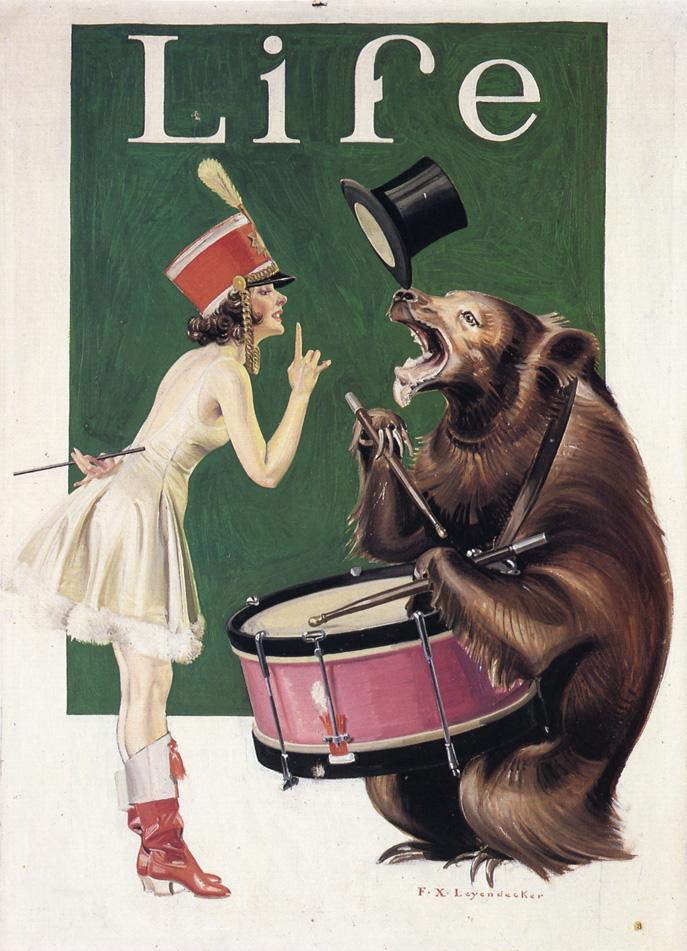The image is a detailed color oil painting in portrait orientation, serving as a magazine cover. At the top, against a green background, the title "LIFE" is prominently displayed in white serif font. Below this title, the scene captures a whimsical moment featuring a circus-themed act. 

On the left side, a young Caucasian woman stands facing a brown bear. She is dressed in an elaborate costume reminiscent of a circus performer: a light yellow dress adorned with a floofy ruffle or fur trim, red high-heeled boots, and a red marching band conductor’s hat, complete with a center feather and gold trim around the chin. Her attire also includes short, curled brown hair. The woman is bent slightly at the waist, leaning forward, with her right arm raised and her finger held up in a shushing gesture, while her left hand, positioned behind her back, holds a conductor's baton.

The bear, positioned to her right, engages actively in the scene, wearing a military-style drum around his neck. He is depicted in the process of playing the drum with drumsticks held in his claws. Adding to the whimsical nature, a black top hat appears to be precariously balanced on or tossed above his nose.

This artwork, entitled "The Bear Trainer" by Frank Javier Leyendecker, is executed in a style consistent with Art Nouveau illustration. The bottom right corner of the image features Leyendecker’s signature, cementing the piece’s authenticity and artistic value.